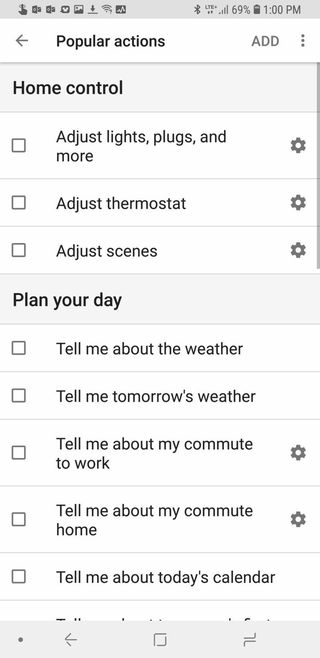The image displays a smartphone screen with various icons and widgets. At the top, the screen shows status information: "Wi-Fi," "Bluetooth," and a battery indicator at "69%." The time displayed is "1 PM."

The screen is filled with categories for "Popular Actions" and options related to "Home Control." Each category has a series of checkboxes beside the respective settings.

- The "Popular Actions" section includes options with checkboxes reading:
  - "Not checked: Adjust lights, plugs, and colors"
  - "Not checked: Adjust thermostat"
  - "Not checked: Adjust scenes"
  - "Not checked: Tell me about the weather"
  - "Not checked: Tell me tomorrow's weather"
  - "Not checked: Tell me about my commute"
  - "Not checked: Tell me about today's calendar"

- Icons such as a gear symbol next to the thermostat adjustment option and a square for the calendar option are displayed.

Below, there is a "Gray bar" that visually separates the sections. The bottom area has dark circles, possibly for navigation or indicating inactive options, with one highlighted, presumably the active section.

All the elements are organized neatly, offering a clear overview of home automation and informational features, awaiting user interaction to personalize the setup.